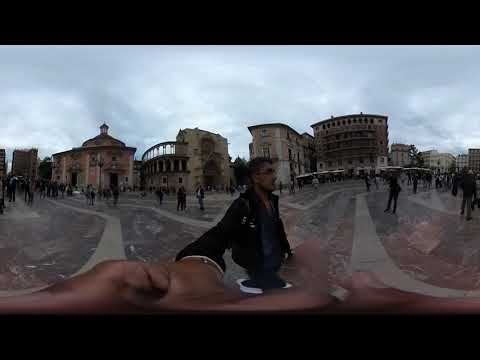A young man with short dark hair and glasses is captured in the center of the image, taking a selfie with his arm stretched out, causing a slight distortion that makes his hand and arm appear elongated. He is dressed in a long-sleeved black jacket and dark blue shirt, with black trousers, standing in what appears to be an open, stone-paved area. The background showcases several old buildings, some of which might be ancient ruins, evoking the atmosphere of a historic tourist attraction. The sky is overcast and gray, adding a somber tone to the scene. The area is bustling with tourists, all dressed in darker colors, walking and exploring the surroundings. The backdrop of the image includes brown and yellow structures, hinting at an ancient city, possibly with a coliseum or similar historical monument. Cars can be vaguely seen in the distant background, emphasizing the location within a city setting. The young man seems to be documenting his visit, possibly live-streaming a tour of the significant sights around him.